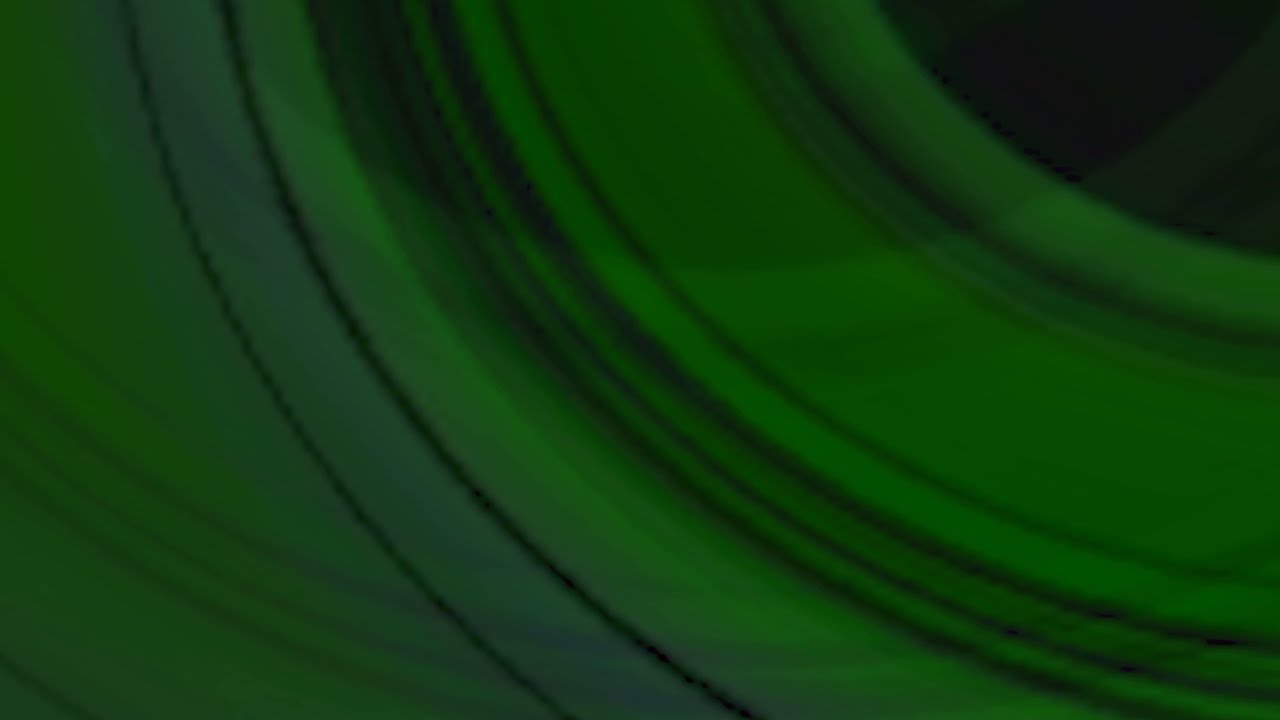This image is a highly detailed, close-up photograph primarily featuring vibrant green hues with intricate grooves and wavy, circular lines that vary in width and texture. The main surface is characterized by a series of alternating raised and indented areas, giving it a textured, non-smooth appearance. The pattern closely resembles overlapping plates or perhaps a plastic object, like a frisbee, viewed up close. The image includes additional colors such as black and hints of blue, which are particularly noticeable in the diagonal, swirling designs that flow across the image. The top right corner reveals a dark, almost black area, possibly representing a shadow or a void. This corner contrasts sharply with the luminous, rich green that dominates the rest of the image. The interplay of light and shadow adds depth and a sense of three-dimensionality to the photograph, enhancing the mesmerizing, almost hypnotic appearance of the green swirl.